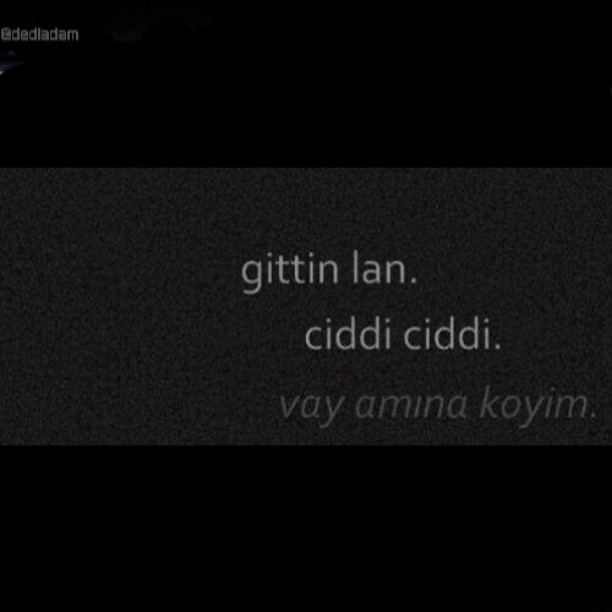The nearly square image features predominantly black sections at the top and bottom, framing a thick, textured, dark gray band in the middle. This middle band resembles a grainy, staticky field, reminiscent of fine sediment. Three lines of text are embedded within this dark gray band. The first two lines are in a light gray, regular font, while the third line is in a slightly darker gray and italicized.

The first line reads "GITINLAN." The second line, positioned slightly to the right, says "CIDDI CIDDI." The third line, italicized, declares "Vaya Amina Koyim." Additionally, at the very top of the image, in the upper left corner of the black section, the handle "DEDLADAM" is subtly visible.